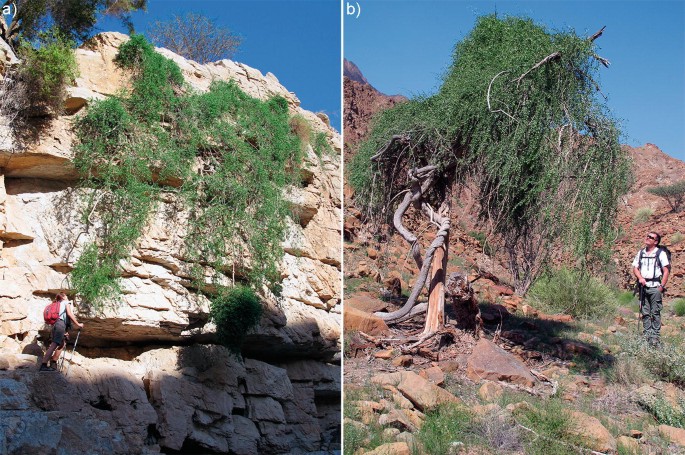The combined image features two photographs of a rugged, rocky hillside, likely from the United Arab Emirates or broader Middle East region. Both images exhibit a canyon-like setting with a steep cliff. In the left image, labeled "A," a hiker is seen near a cliff where a tree with long strands of leaves, resembling a weeping willow though more likely a sandalwood tree, has grown out of the side and extends downwards. The cliff possesses a stark contrast of beige and brown hues, adding to the rugged aesthetic. In the right image, labeled "B," the same type of tree is shown growing upward normally with elongated branches and tiny leaves cascading elegantly. The scene is set against a backdrop of a rocky mountainside, emphasizing the harsh yet beautiful terrain where hikers with backpacks explore the sandstone formations.